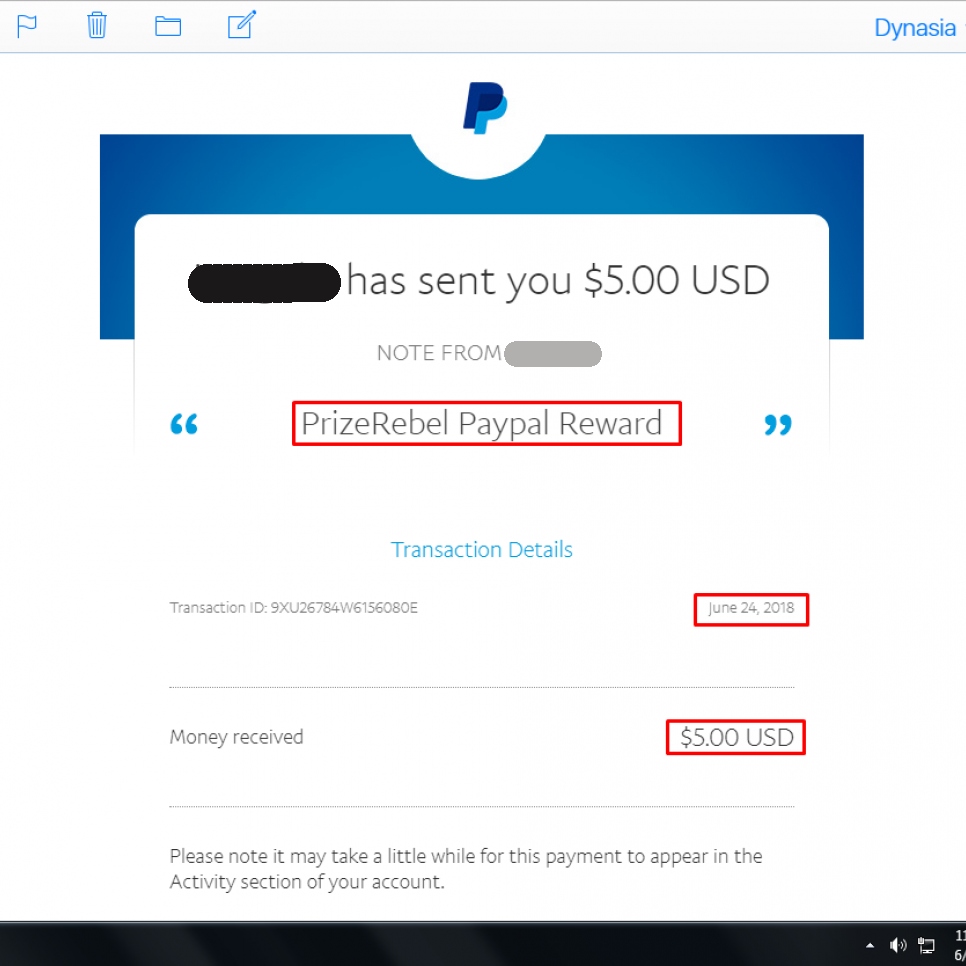Screen capture of a PayPal transaction on a web page. At the top, there is a ribbon featuring several icons: a flag, a trash can, a folder, and a pencil inside a square. The center of the screen prominently displays the standard PayPal logo. Below the logo, the sender's name has been obscured. The text to the right reads, "has sent you $5 USD." Further below, there's a section labeled "Note from [Name Redacted]," with the note reading "Prize Rebel PayPal reward" highlighted by a red rectangle.

Detailed transaction information follows: 
- The transaction ID number (not fully visible in this description).
- The date, "June 24th, 2018," also highlighted in red.
- The amount received, "$5 USD," similarly highlighted in red.

At the bottom, a note indicates that the payment may take some time to appear in the account's activity section. In the upper right corner of the screen, the name "DYNASIA" is visible, presumably the name of the account owner or the person who took the screen capture. The purpose of this screen capture appears to be for documenting the sender, the date, and the amount of the PayPal transaction.